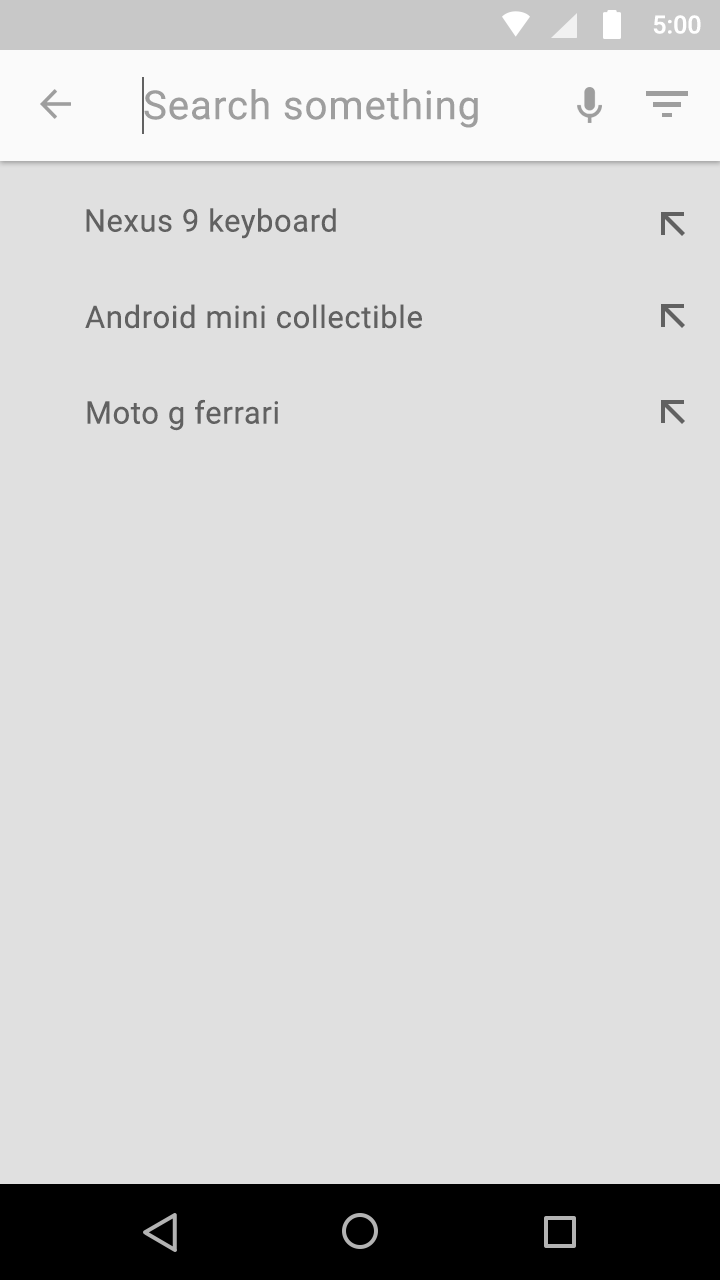The screenshot features a user interface with a predominantly gray and white theme. At the top, a white horizontal banner spans the entire width of the page, containing various gray elements. On the left, there's a gray arrow indicating a back function. Next to it, the words "Search something" are displayed in gray text. Adjacent to this, on the right side, there are two icons—one of a microphone and the other representing a menu—both in gray.

Below this banner, a large gray square occupies most of the screen. At the top of this gray section, in black text, the phrase "Nexus 9 keyboard" is prominently displayed, accompanied by a black arrow pointing to the upper left. Beneath this, another label, "Android Mini Collectible," is similarly styled with a black arrow pointing to the upper left. Further down, the text "Moto G Ferrari" is shown, again with a black arrow pointing to the upper left.

The bottom of the screen contains menu options set against a black background, though the specific icons or text within this menu are not detailed in this description.